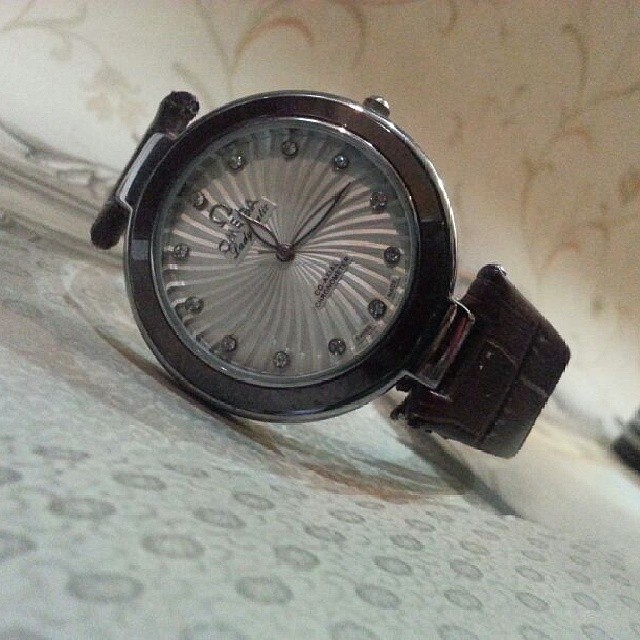This image depicts a partial view of an elegant Omega wristwatch, emphasizing its intricately designed face and luxurious details. The watch, adorned with silver studs in place of numbers, has a striking spiral pattern resembling a vortex, accentuated by a combination of white and silver hues. Its silver rim adds to the sophistication, while the small silver knob on the side further enhances its refined appearance. The wristband, which is partially visible, appears to be made of brown leather. The watch is positioned on a surface that suggests light gray and white floral patterns, casting a subtle shadow against it. In the background, there is a white wallpaper featuring delicate brown leaf-like designs, enriching the visual texture of the scene.